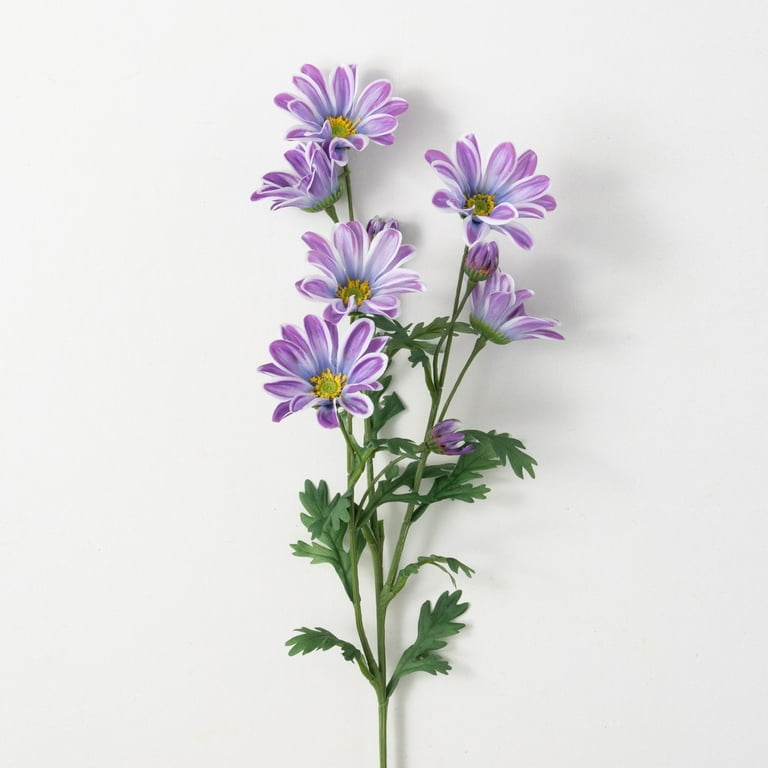The image shows a realistic twig with dark green leaves reminiscent of parsley, placed centrally against a plain, white painted wall. The stem supports a series of vibrant flowers, each with a yellow center and delicate petals that transition from white at the base to a light purple at the tips. There are about six fully bloomed flowers and three buds in various stages. The floral arrangement, featuring petals with numerous serrated edges, provides a soft, yet striking visual contrast against the white background, creating an effect that makes it challenging to discern if the flowers are real or illustrated.